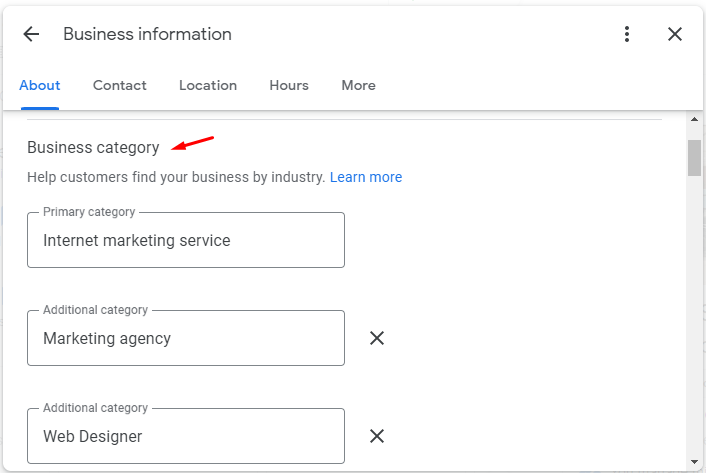The web page features a minimalist design with a plain white background. At the top left corner, "Business Information" is displayed in unadorned, simple text. An arrow pointing to the left is present, accompanied by three dots and an 'X' on the right side. Below this header, the menu options "About," "Contact," "Location," "Hours," and "More" are listed, with "About" prominently highlighted in blue and underlined.

In the midsection, extending towards the bottom, the section labeled "Business Category" is marked by a red arrow indicating its importance. A prompt underneath reads "Help customers find your business by industry," and a clickable "Learn more" link in blue is situated next to it.

The "Primary Category" field is enclosed in a gray box, identifying the business as an "Internet Marketing Service." Directly below, another gray box labeled "Additional Category" lists "Marketing Agency," with an 'X' for removal on its right. Similarly, another "Additional Category" with "Web Designer" is presented, also featuring an 'X' for deletion.

On the right side, a large gray section includes a darker gray scrollbar, indicating the presence of additional content that can be accessed by scrolling. The webpage remains stark and utilitarian, ensuring functionality over aesthetics.